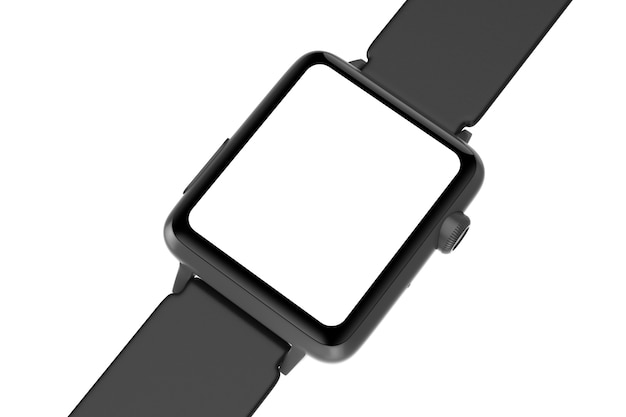This image showcases a sleek, minimalist watch with a prominent blank, white face where the dial would typically be, suggesting it may be a product placeholder or a composite mock-up. The watch features a smooth, solid black band without ridges or holes, extending from the upper right to the bottom left of the frame. The watch's frame is also black, seamlessly matching the band and enhancing its monochromatic aesthetic. There is a small knob on the right side of the watch face and a button on the left side. The background is stark white, creating a contrasting backdrop that highlights the watch's dark gray and black tones. This simple, uncluttered setting emphasizes the watch's clean design and potential as a versatile accessory.